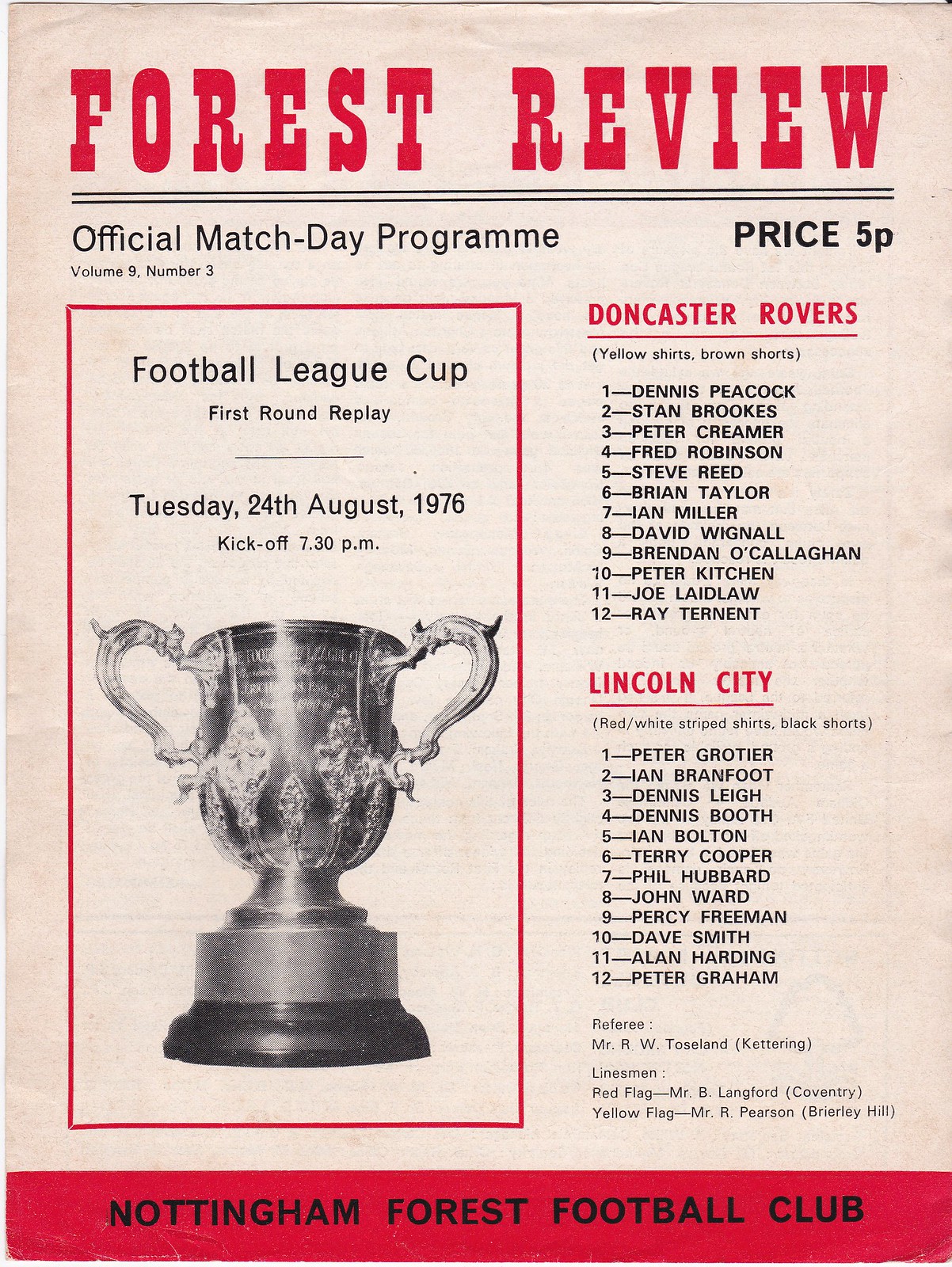The image depicts an aged and slightly browned cover of a soccer program titled **"Forest Review."** The cover features red letters prominently at the top stating **"Forest Review"** and beneath a dividing bar, the text **"Official Match Day Program, Volume 9, Number 3"** along with the price **"5P."** Below a red banner, an illustration of a cup trophy is shown, labeled **"Football League Cup First Round Replay, Tuesday, 24th August 1976, kickoff 7.30pm"** in red text. Playing in the match are **Doncaster Rovers** and **Lincoln City,** with the respective player rosters listed for each team, both in black text. The referees and linesmen’s names are mentioned: Referee **Mr. R.W. Towsland from Kettering;** Linesmen **Langford, Pearson from Coventry, and Briar-Lay Hill.** The details are meticulously organized, with the names **Doncaster Rovers** in red and the list of twelve players, followed by **Lincoln City** and its roster, also detailed in red and black text. Concluding the cover, the bottom features the words **"Nottingham Forest Football Club"** in red banner text.